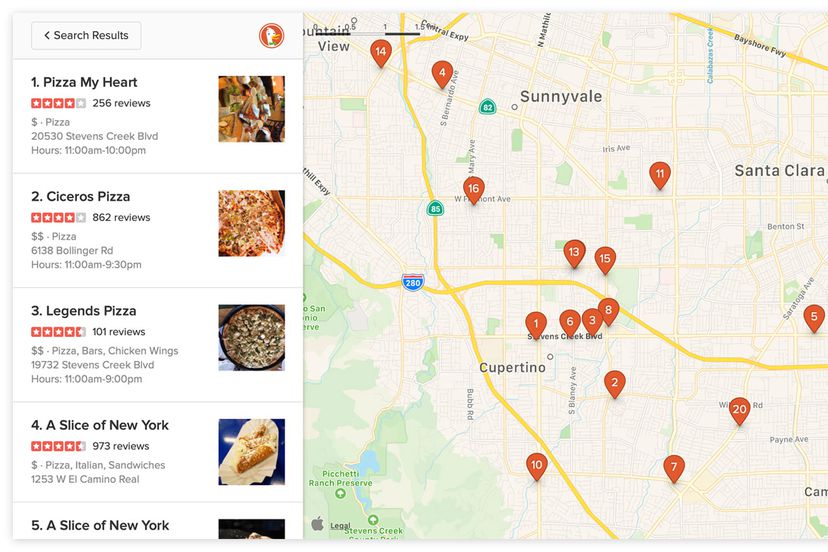An image of a DuckDuckGo search engine map page prominently displays a navigational layout for locating pizza places. On the left-hand side, there's a sidebar featuring a search bar at the top, accompanied by the DuckDuckGo logo to its right. Within the search bar, the term "search results" is visible. Below the search bar, there is a detailed list of various pizza establishments. Each listing is accompanied by photographs on the right and descriptions on the left. Notable pizza places listed include Pizza My Heart, Cicero's Pizza, Legends Pizza, and A Slice of New York. To the right of the sidebar, a map is showcased, pinpointing the exact locations of all the mentioned pizza venues.